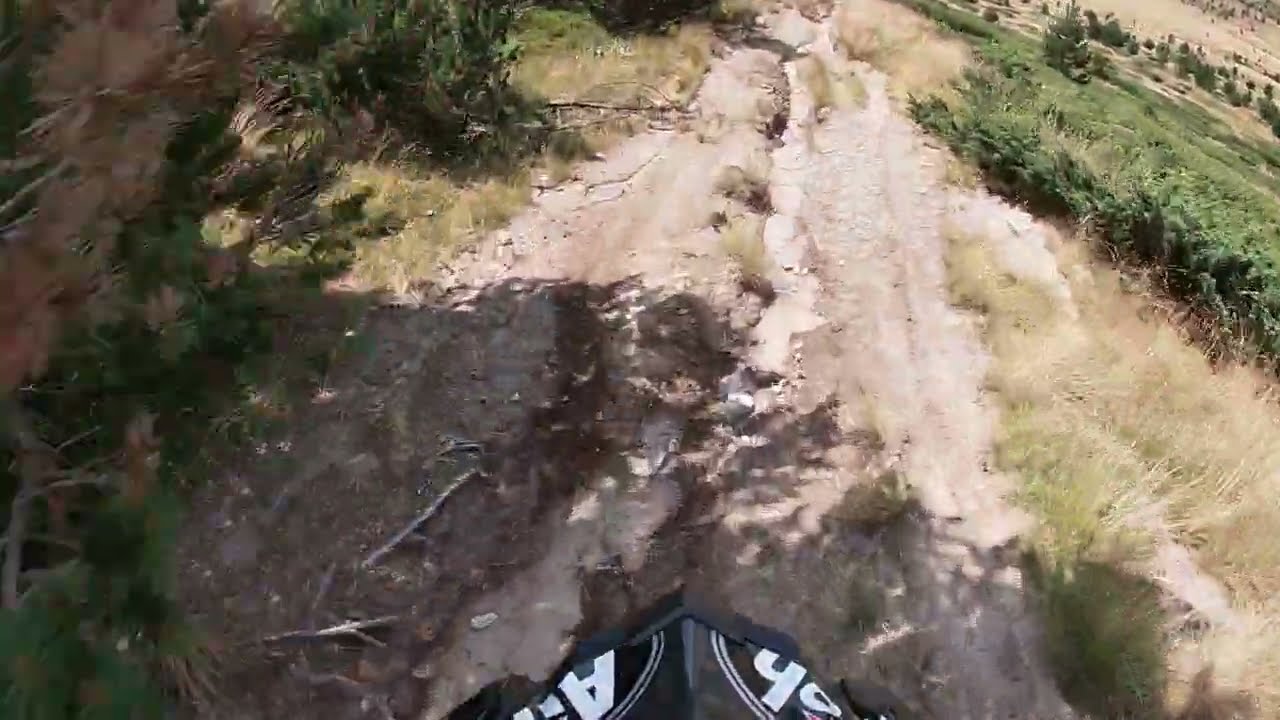This photograph appears to be taken from a GoPro camera mounted on a cyclist's helmet. The very brim of the black helmet with illegible white lettering is visible at the bottom center of the image. The scene captures a rugged dirt path with a deep rut running down its center, likely formed by water erosion. On either side of the path, there is tall, yellowish-green grass interspersed with shrubs. In the foreground, on the left side of the image, there are pine trees with a dense covering of needles. The day appears sunny, casting scattered shadows across the path and surrounding vegetation. The perspective, combined with the helmet's appearance, strongly suggests the photographer is biking down this uneven path. The surroundings include a mix of green foliage and brown dirt, creating a natural, untamed setting.